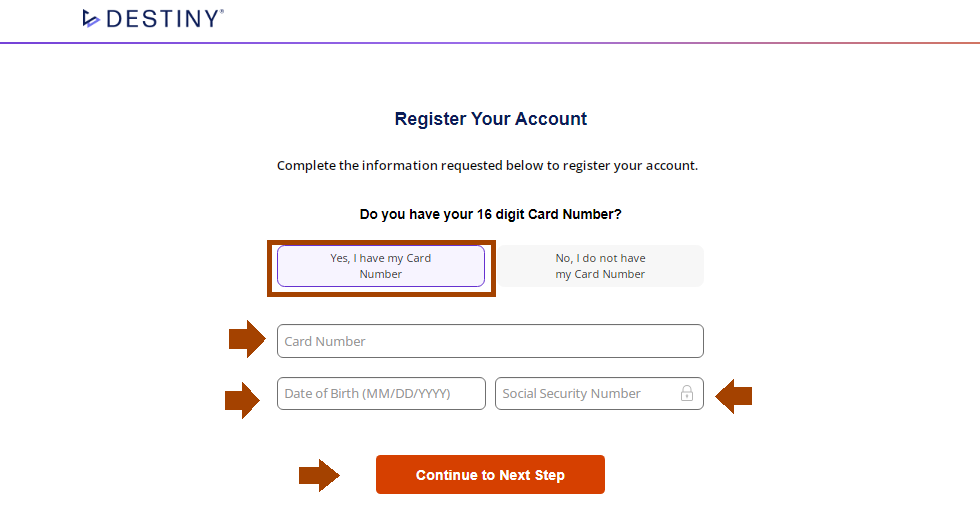This screenshot captures the homepage of a website called "Destiny," prominently displayed in the top left corner in a dark blue font, accompanied by the company logo. The logo features two arrowhead-shaped bullet points—one in blue and the other in light purple—pointing to the right. Just beneath the title "Destiny," a line stretches across the page, transitioning in color from medium blue to pink as it progresses.

Immediately following the line, large blue text instructs users to "Register Your Account." Subtext below the heading elaborates: "Complete the information requested below to register your account." The page first prompts users with a highlighted question: "Do you have a 16-digit card number?" Users must select between two options: "Yes, I have my card number," or "No, I do not have my card number." The form requires the card number or alternative information to proceed. Once the necessary details are entered, users can click an orange "Advance" button to move to the next step.